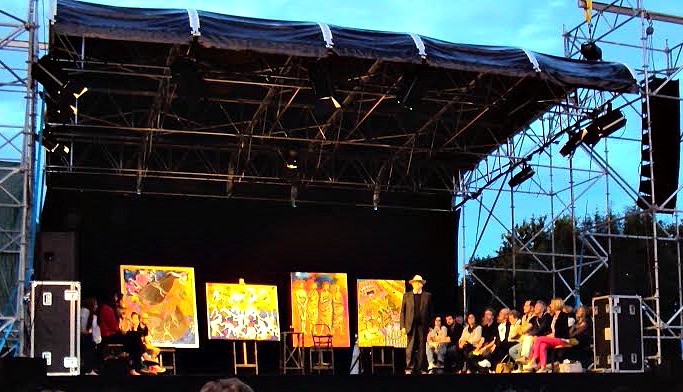An outdoor stage, covered by a black canopy and framed with extensive scaffolding on the sides and ceiling, stands illuminated under a darkening sky that hints at dusk. The stage, with its black backdrop, is set for what appears to be an art exhibition. In the center, an older gentleman, distinct in his tan fedora, grey jacket, black shirt, and grey pants, faces the camera. Behind him, four vibrant paintings portraying human figures in warm tones of orange, yellow, and white are displayed on easels. A small table with a drink and a stool sits nearby, further accentuating the scene. The left and right sides of the stage host seated individuals, with noticeably more people on the right, arranged in two or three rows. The stage is cluttered with various pieces of equipment, possibly speakers and railings, contributing to the setup. The overarching view suggests the perspective of an audience member, observing this captivating fusion of art and performance under the early evening sky.